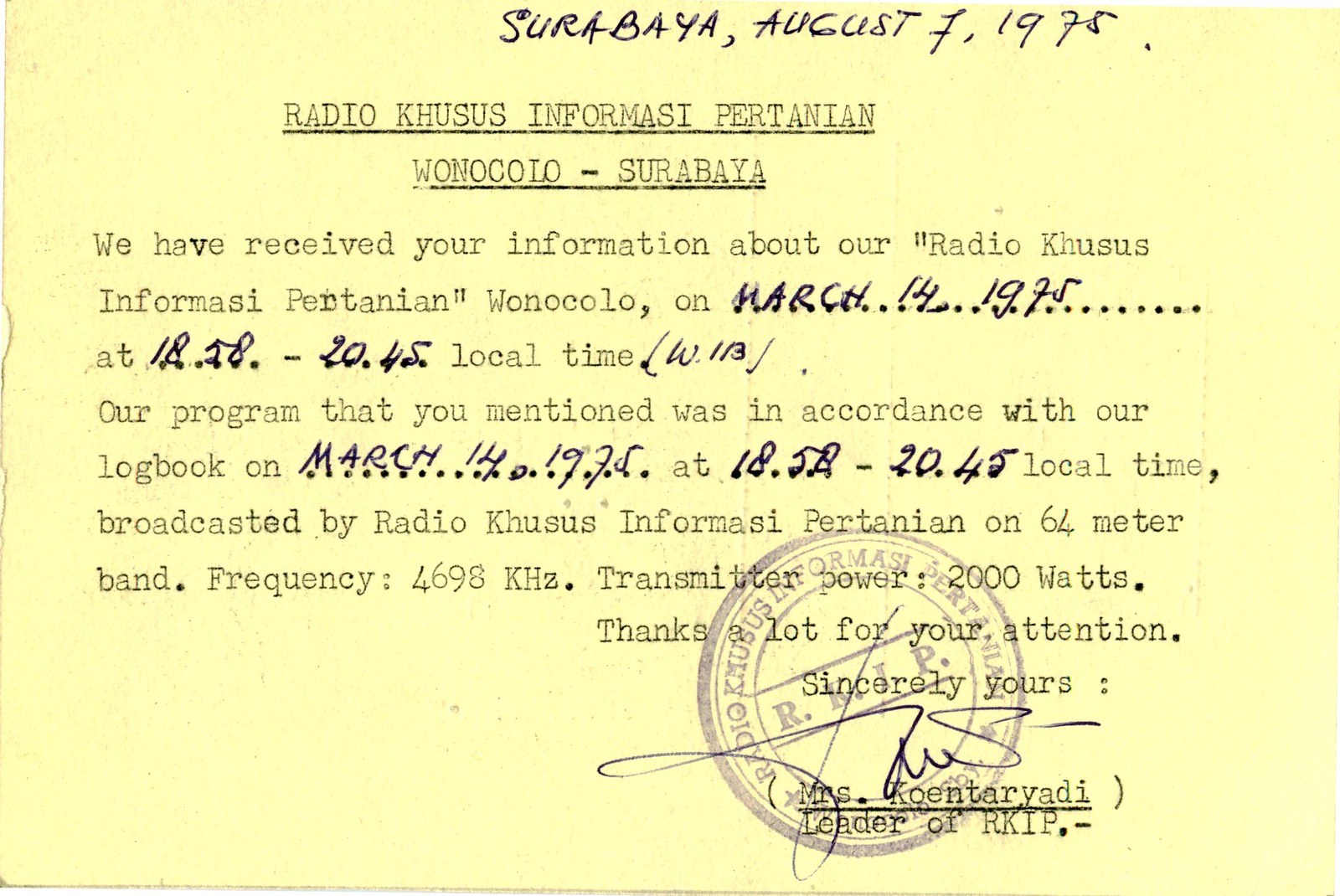The image depicts a yellow rectangular piece of paper with a handwritten inscription at the top reading "Surabaya, August 7, 1975" in black ink. Below this, in typewritten text, it reads: "Radio Cusus Informasi Pertanian, Guanapolo-Surabaya." This heading is underlined. Following this, the message states: "We have received your information about our 'Radio Cusus Informasi Pertanian, Guanapolo,'" and continues, "on March 14, 1975, at 1858-2045 local time." Notably, the time and the date are annotated in black ink. Alongside the time, the notation "(W. 113)" appears in parentheses. The message also indicates that the program mentioned aligns with their logbook records. Near the end, specific broadcast details are provided: "64 meter band, frequency 4,698 kilohertz, transmitter power 2,000 watts." The letter concludes with a note of gratitude, "Thanks a lot for your attention," and is signed, "Sincerely yours, Ms. Koontara Yadi," the leader of RKIP. This signature is handwritten in black ink.